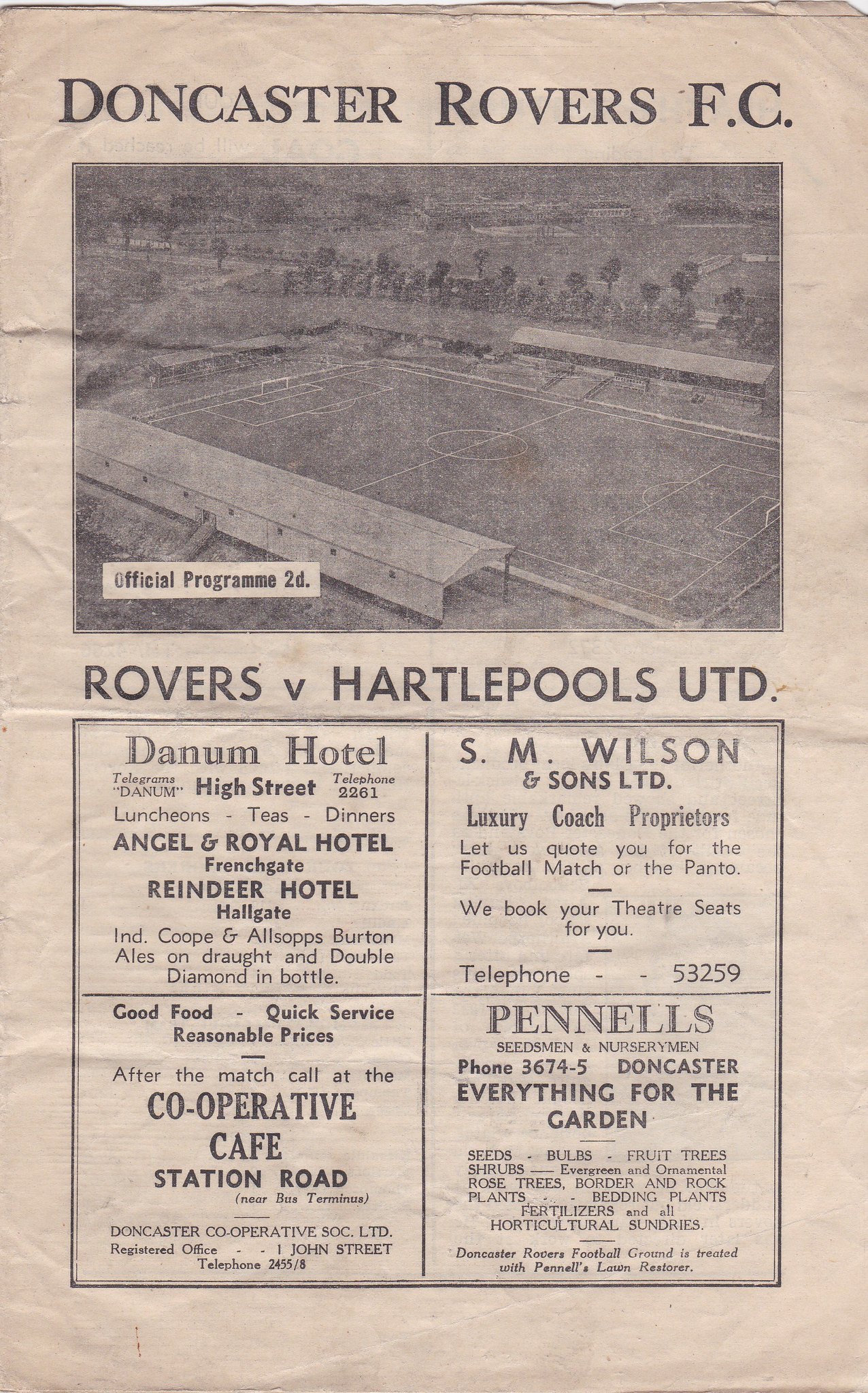The image resembles an aged, beige-tinted newspaper clipping titled "Doncaster Rovers F.C." at the top. Beneath the title is a black and white photograph of a soccer field. Directly under the photograph is another heading: "Rovers vs. Hartlepools UTD." The paper displays the text "Official Programme 2D" in the bottom right corner of the photograph. Further down, there are four distinct advertisement boxes. The top left box advertises "Denham Hotel," with noted services including luncheons, teas, dinners, featuring a telegram and phone number for reservations. The top right box features "S.M. Wilson and Sons Ltd," highlighting luxury coach services for football matches and theater bookings, along with their contact information. The bottom left box promotes good food with quick service at "Co-operative Cafe," providing its location and phone number. The bottom right box presents "Panels," detailing various horticultural supplies like seeds, bulbs, shrubs, and fertilizers, and includes their contact number. The overall layout portrays various font styles and sizes, enveloped in a vintage sepia tone that enhances the nostalgic feel of the piece.